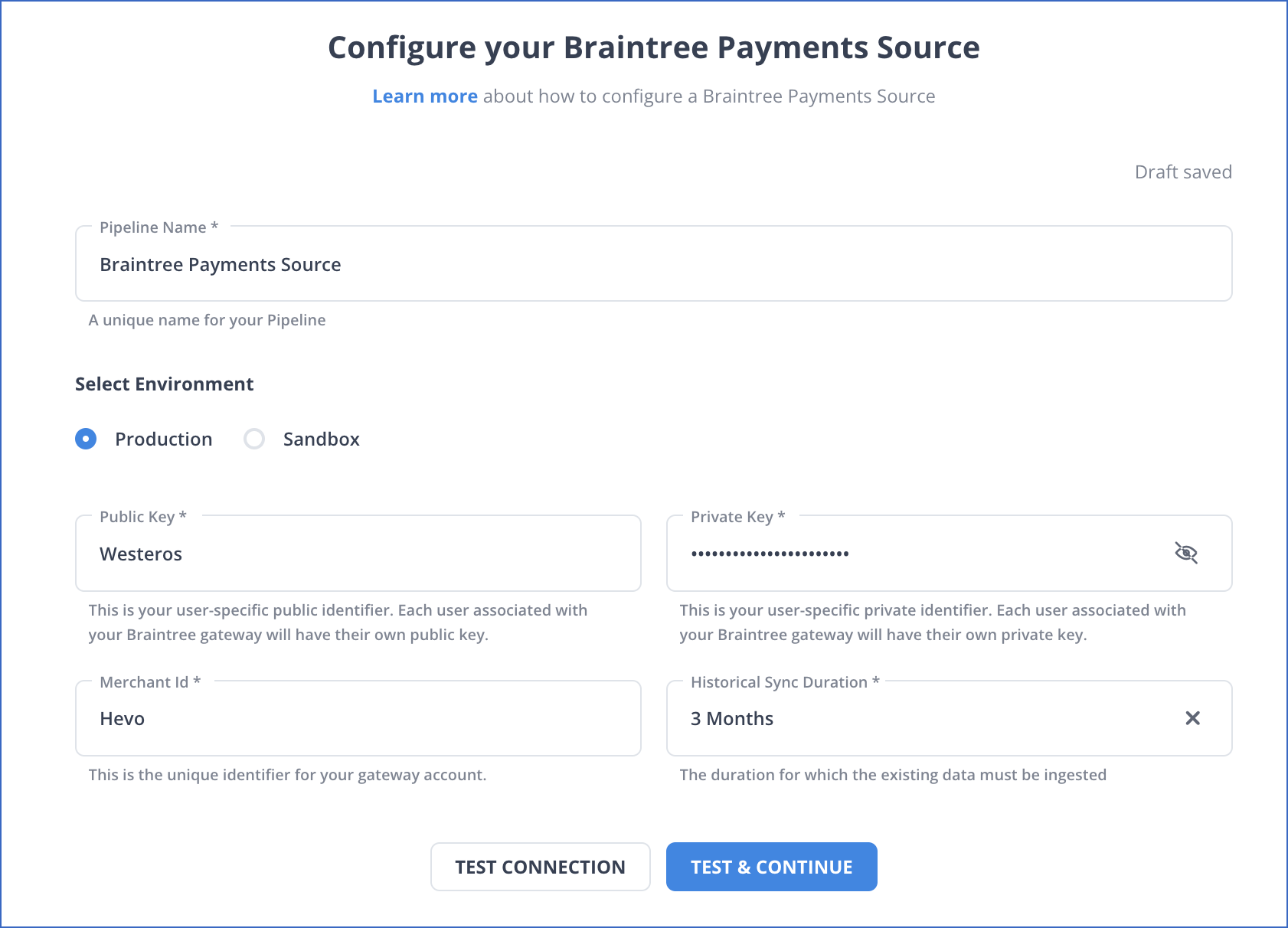This is an image of a webpage dedicated to configuring a Braintree payment source. At the top, a notification states "Draft saved." Below that is a section titled "Pipeline Name" with the provided name "Braintree Payment Source" and a description that reads "A unique name for your pipeline."

The next section allows users to "Select Environment," offering the options "Production" and "Sandbox," with the "Production" option selected. Following this, there are fields for "Public Key" and "Private Key." The public key field contains the placeholder "Key Westeros," while the private key shows masked characters, likely representing a password.

Subsequently, there is a "Merchant ID" field associated with a "Historical Sync Duration" set to "Three months." 

The page also features "Test" and "Test and Continue" buttons for functionality testing. Detailed information is provided under the Public Key, Private Key, and Merchant ID fields, explaining their purposes:

- Under "Public Key," it reads: "This is your user-specific public identifier. Each user associated with your Braintree gateway will have their own public key."
- Under "Private Key," it states: "This is your user-specific private identifier. Each user associated with your Braintree will have their own private key."
- Under "Merchant ID," the text specifies: "This is the unique identifier for your gateway account."

Lastly, the description for "Historical Sync Duration" clarifies it as "The duration for which the existing data must be ingested."